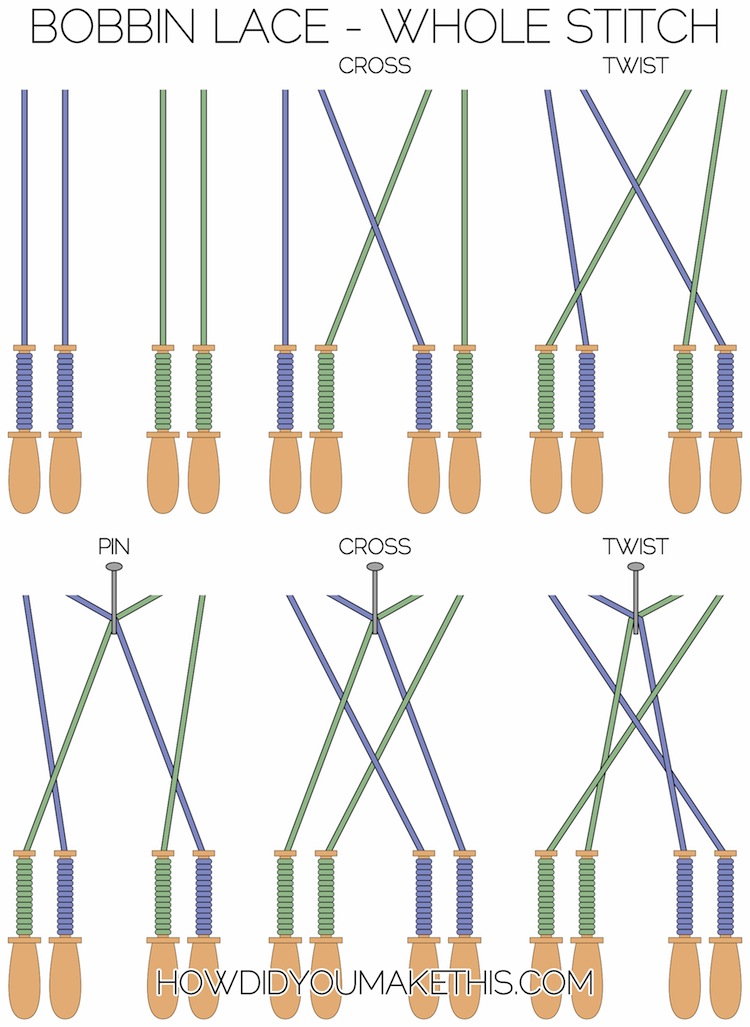The graphic image is a vertical rectangular chart with no external border, designed to demonstrate various sewing techniques for creating bobbin lace using the whole stitch method. The background is white, and the chart is titled at the top in black letters: "bobbin lace - whole stitch, cross, and twist". 

The main section of the image features several illustrations depicting wooden pins or bobbins, which resemble shish kebab skewers or screwdrivers, with each pair wrapped in green and blue threads. The diagrams show different stages of the technique, including crossing and twisting the threads in specific patterns: blue-green-blue-green, with some threads crossing over each other at various points. 

In the bottom left corner, there are additional instructions: "pin, cross, and then twist again". The text is further accompanied by a watermark at the bottom center of the image, which reads "howdidyoumakethis.com" in black letters. The image is presented in a clear, cartoon-style format to visually guide the viewer through the sewing process.